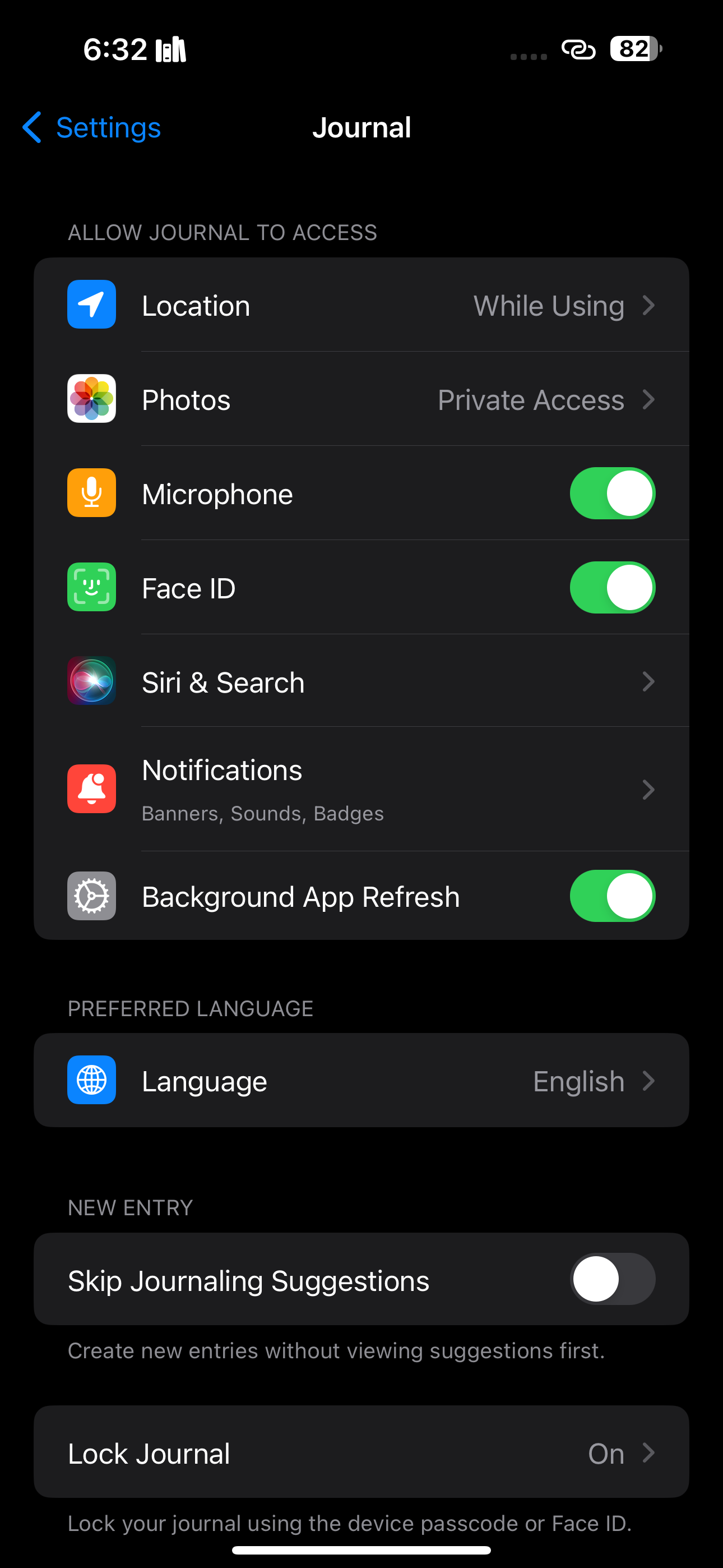The image displayed is a screenshot of a cell phone screen. The time shown on the upper-left corner is 6:32, and on the upper-right corner, the battery level is at 82%, accompanied by a chain-like hyperlink symbol. The screen is on a page titled "Journal," which appears to be an application.

Below the title, there is a section labeled "Allow Journal to Access," indicating the app permissions required. The listed permissions include:

- **Location:** Set to "While Using" the app.
- **Photos:** The access level is set to "Private Access."
- **Microphone:** The toggle switch is turned on.
- **Face ID:** The toggle switch is also turned on.

Further down the screen, there is a heading for "Siri & Search," followed by a forward arrow indicating additional options available upon selection. Underneath this is a section for "Notifications," which shows options for "Banners, Sound, Badges."

Continuing to the next section, "Background App Refresh" is checked off. The language setting is marked as "English," and the option for "Skip Journaling Suggestions" is toggled off.